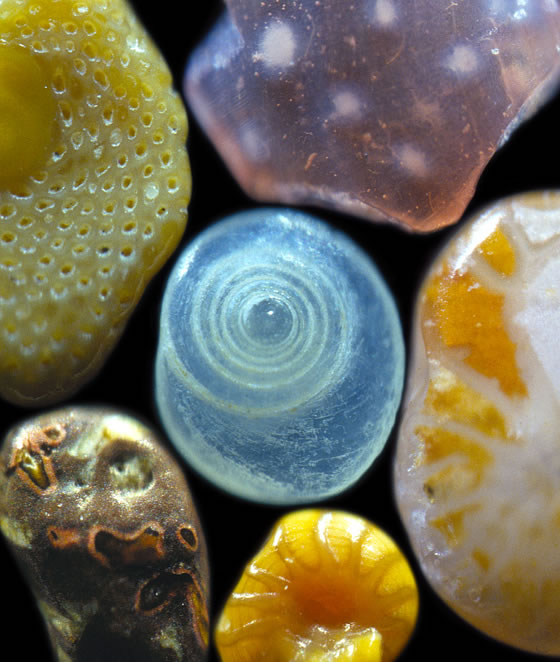The image is a highly magnified photograph showcasing six abstract, circular objects with uneven edges, making them appear blob-like. These objects vary in color and texture, evoking comparisons to both sea creatures and inanimate items like rocks or candy. The central object is a swirling blue shape that looks reminiscent of a tornado or cyclone. In the top right corner, there's a clear, translucent blob that could be likened to a jellyfish. A yellow object with small perforations resembles the texture of a strawberry and sits prominently in the scene. Another white object features bits of gold-yellow and looks almost like a disfigured peppermint due to its uneven coloration. At the bottom, a striped gold object resembles a cartoon cat's tail. Lastly, a brown object with orange flecks appears shiny and metallic. The overall composition is colorful and varied, capturing the viewer's attention through its intricate details and mysterious forms.